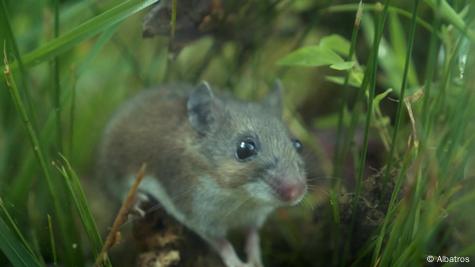In this detailed, zoomed-in image captured in nature during daytime, a small furry creature—likely a shrew or a mouse—takes center stage amidst a backdrop of green plants, dirt, and possibly some tree debris. The animal, with its distinguishing gray back, white underbody, and pink claws, features the characteristic black beady eyes, a pink nose, and larger ears which may appear slightly pulled back. It sits on a dark rock, surrounded by blades of grass that tower over its diminutive size. The background includes additional green foliage, twigs, and what seems to be part of a tree log or a crumpled leaf. In the bottom right corner, there is a small white text that reads "copyright albatross".